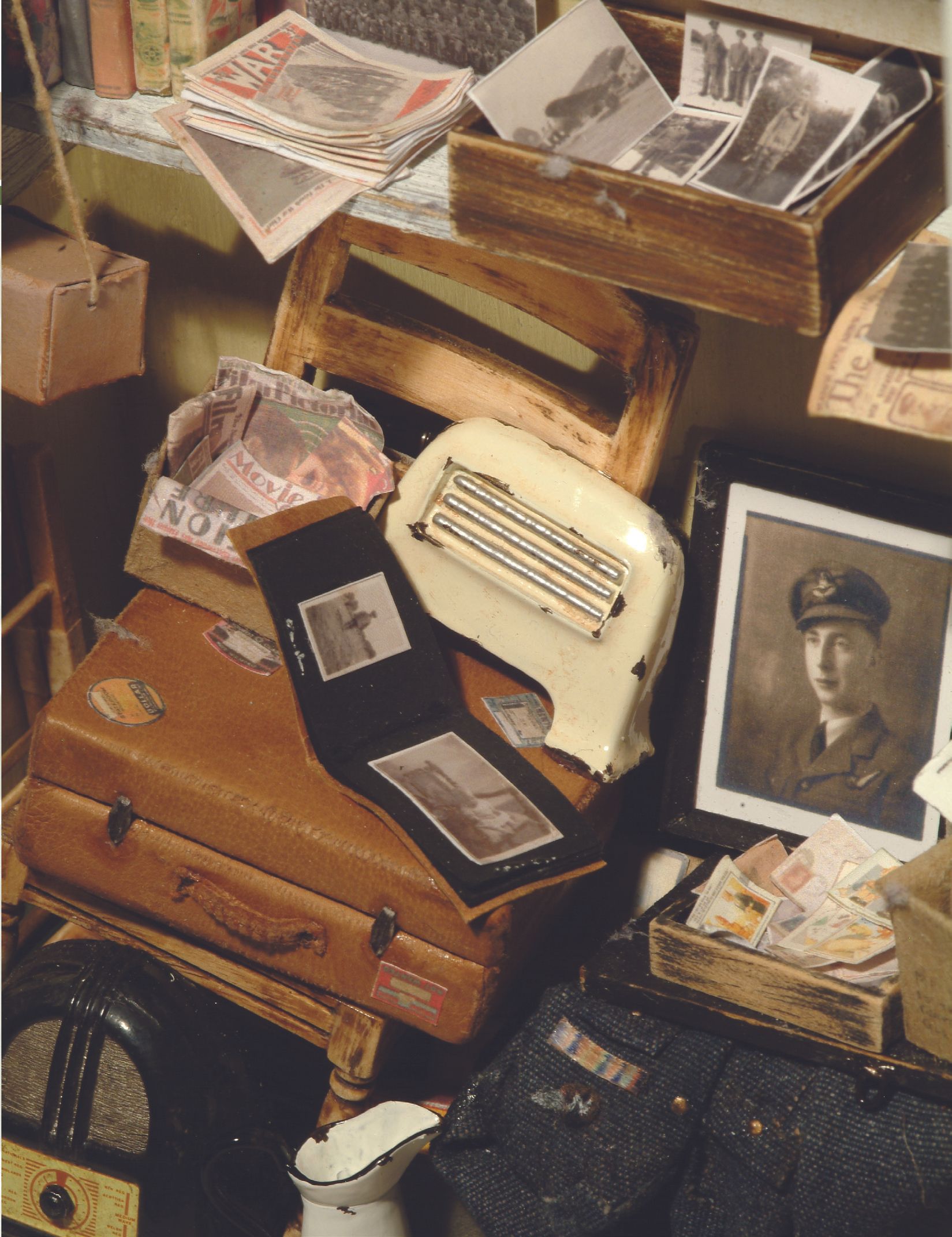This image depicts a cluttered scene in what appears to be an antique store, characterized by its vintage and aged items, predominantly in tones of brown and beige. At the top, a wooden box overflows with old black and white photographs, evoking memories of bygone eras. To the left, atop a stack of yellowed newspapers, a headline in faded red and beige letters ominously proclaims "War." Below this collection, an aged leather suitcase adorned with travel stickers stands out. On top of the suitcase rests a small, worn photo album with a brown exterior and black pages, each affixed with black and white portraits. A striking image of a Caucasian man in a military uniform—with a hat, dark tie, and light shirt—captures attention on the right side of the composition. The man’s serious expression matches the somber tone of the image. Further highlighting the vintage theme, an oval-shaped black radio with a single knob is situated in the lower left-hand corner. The entire setting, including various other small objects scattered about, emanates a sense of nostalgia and historical significance, encapsulated in a dusty, yellowed ambiance that suggests a mid-20th-century time frame.